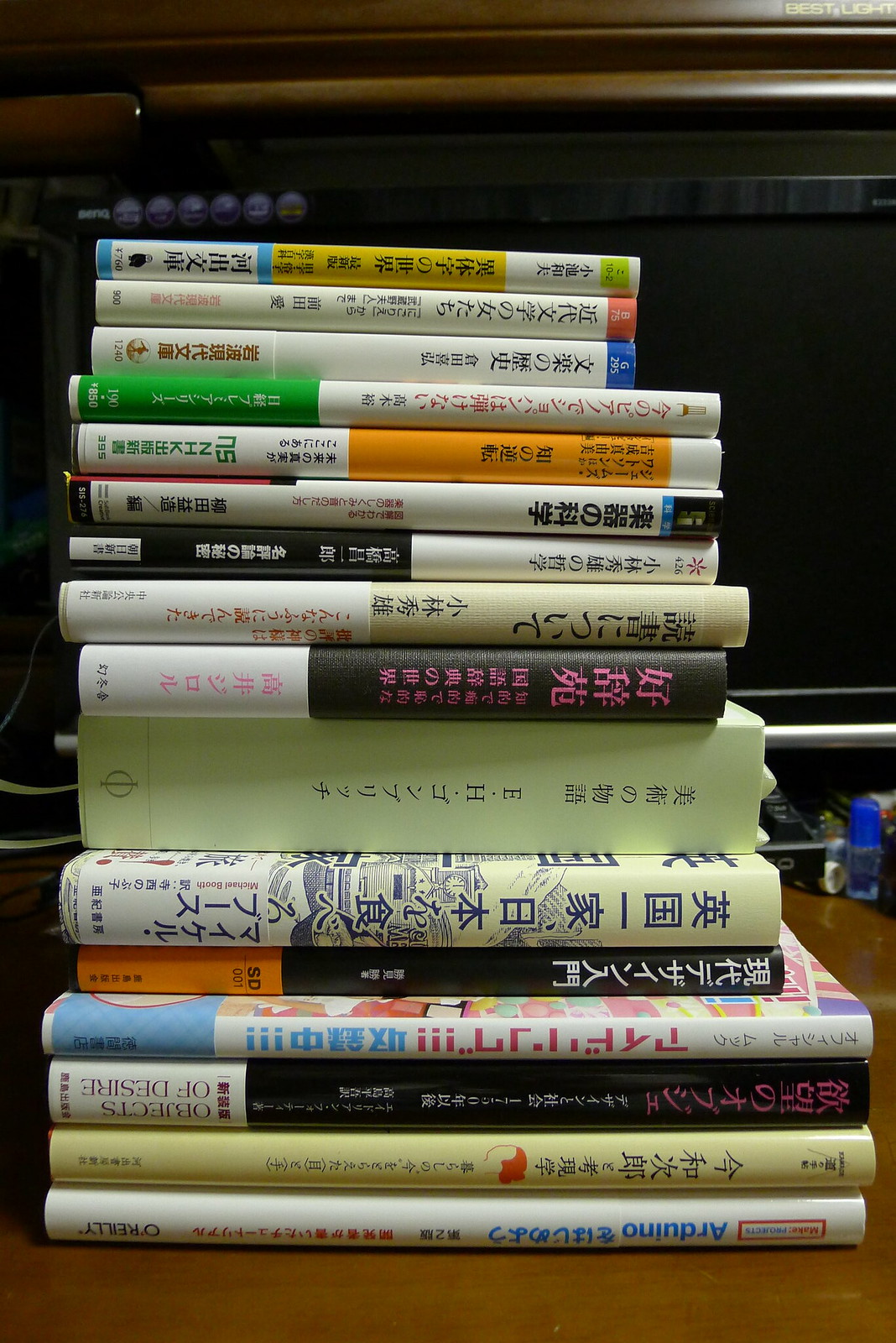A detailed image of a stack of 16 books, written in either Japanese or Chinese, arranged from the largest at the bottom to the smallest at the top. The spines, which are facing forward, feature a variety of colors and thicknesses, denoting both hardcovers and softcovers. The bottom book is predominantly white with a blue side, followed by books of various colors including tan, black, green, orange, and several shades of white and yellow. One book has English text reading "Objects of Desire," while another mentions the printer name "O'Reilly." They rest on a richly colored, dark brown wood table. The background is primarily black, suggesting either a blackboard or a TV screen with circular stickers on its frame. The books' position varies slightly, contributing to an orderly but imperfect stack, reflecting their varied thicknesses and widths. The overall setting is indoors, with a hint of additional objects possibly visible beyond the stack.